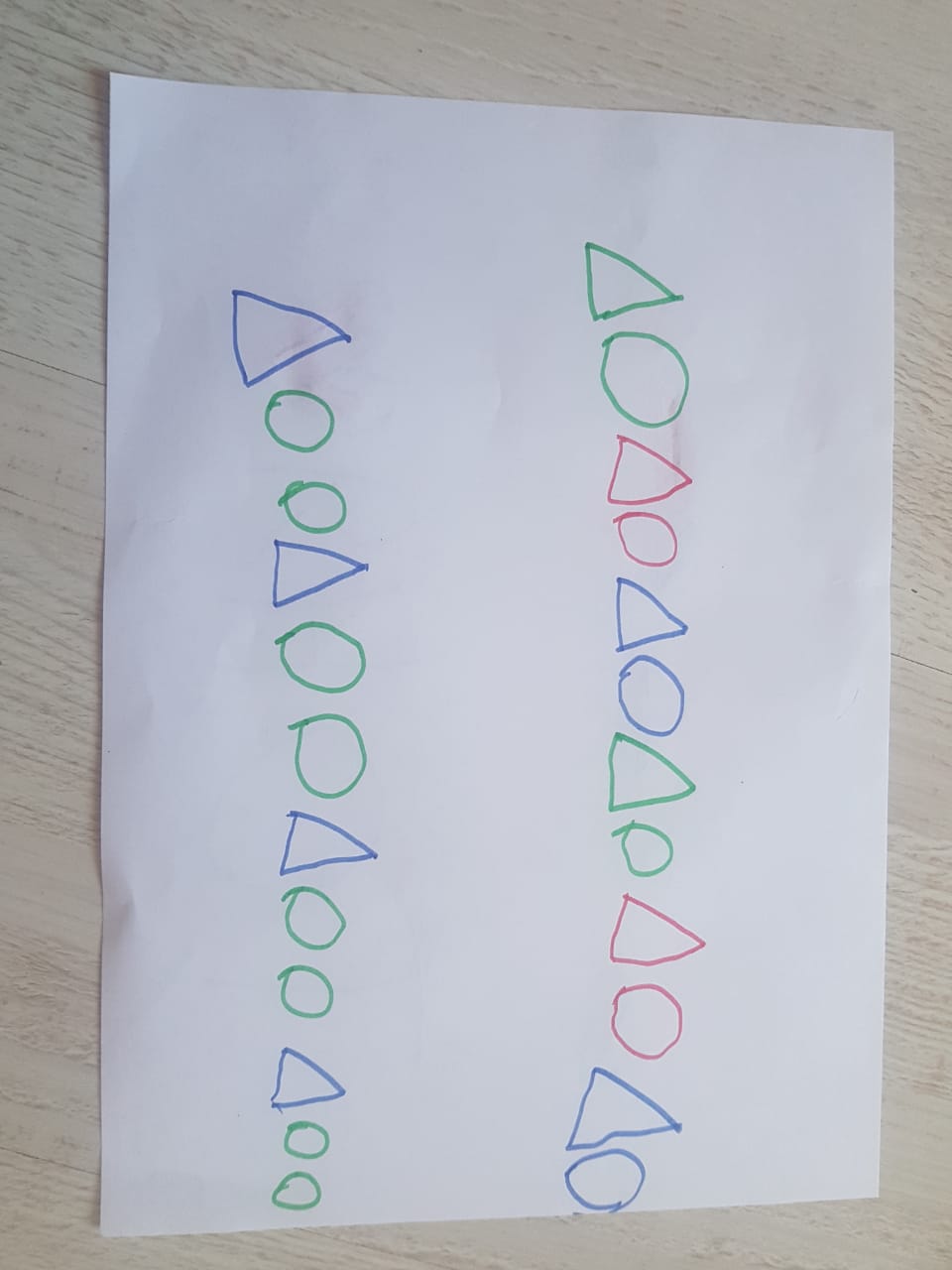In this image, a white piece of paper rests on a light-colored wooden table. The paper features what appears to be a child's drawing, characterized by its playful and imperfect shapes. Starting about a tenth of the way down, the drawing displays two parallel columns composed of various geometric outlines, seemingly drawn with fine-tipped markers.

In the left column, a repeating pattern begins with a blue outline of a triangle, followed by two green circles, and this sequence continues with another blue triangle followed by two more green circles. This pattern repeats multiple times along the column.

On the right column, a similar structure is evident but with a more varied color scheme: it starts with an outline of a green triangle followed by a green circle, then a red triangle and a red circle, and continues alternating with blue triangles and circles as well. These shapes also repeat in a sequence down the column.

None of the shapes are filled in; they are solely outlined in their respective colors. The overall effect suggests a simplistic and charming drawing, likely created by a young child exploring basic shapes and colors with markers.